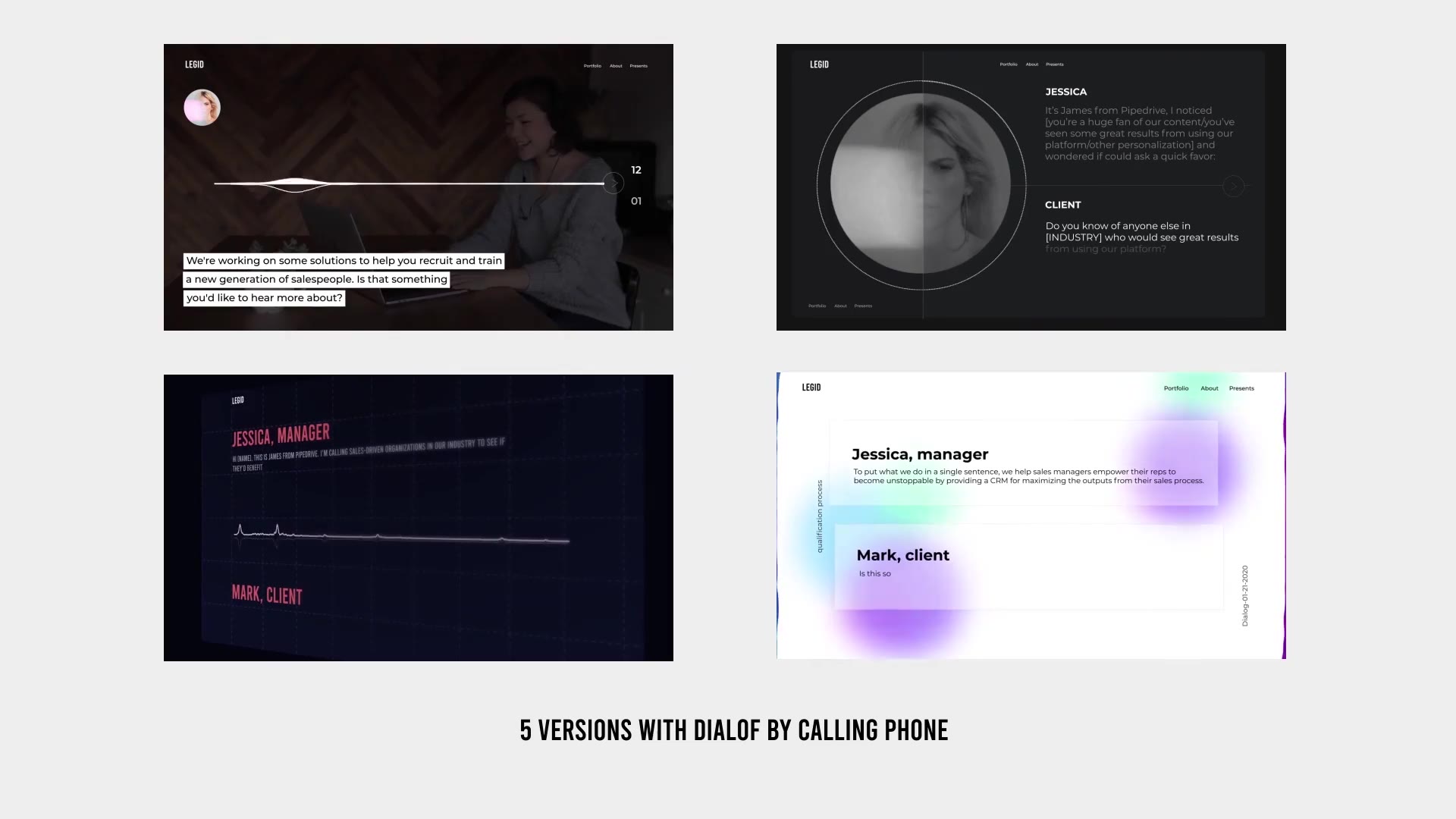The image consists of four distinct screenshots arranged in a square format on a light blue background, each featuring the "Legio" logo in the upper left corner. Here is a detailed breakdown of each screenshot:

1. **Top Left Image**: This screenshot depicts a woman engaged in a video chat on a laptop, positioned before her. The accompanying text says, "We're working on some solutions to help you recruit and train a new generation of salespeople. Is that something you'd like to hear more about?"

2. **Top Right Image**: A monochromatic portrait of a woman, presumably Jessica, is partially obscured by a bright circular light. The text reads, "Jessica, it's James from Pipedrive. I noticed you're a huge fan of our content. You've seen some great results from using our platform [other personalization]. I wondered if I could ask a quick favor. Do you know of anyone else in [industry] who would see great results from using our platform?"

3. **Bottom Left Image**: This screenshot features a tilted angle of a conversation represented by a horizontal sound bar. The dialogue is between "Jessica, Manager" (highlighted in red) and "Mark, Client." However, the text under "Jessica, Manager" is blurry and illegible. The clear portion of the text indicates that Jessica is conversing with Mark.

4. **Bottom Right Image**: This image combines a primarily white background with splashes of light blue and purple. The text at the top reads, "Legio" on the top left and "Portfolio, About, Presence" on the top right. It states "Jessica, Manager" along with, "To put what we do in a single sentence, we help sales managers empower their reps to become unstoppable by providing a CRM for maximizing the outputs from their sales process." The segment attributed to "Mark the client" reads, "Is this so?" Additionally, text on the left indicates "Qualification Process," while the right side notes "Dialogue-01-21-2020."

At the bottom of the image, there is a textual note that reads, "Five versions with dial-off by calling phone," though its purpose and meaning remain unclear.